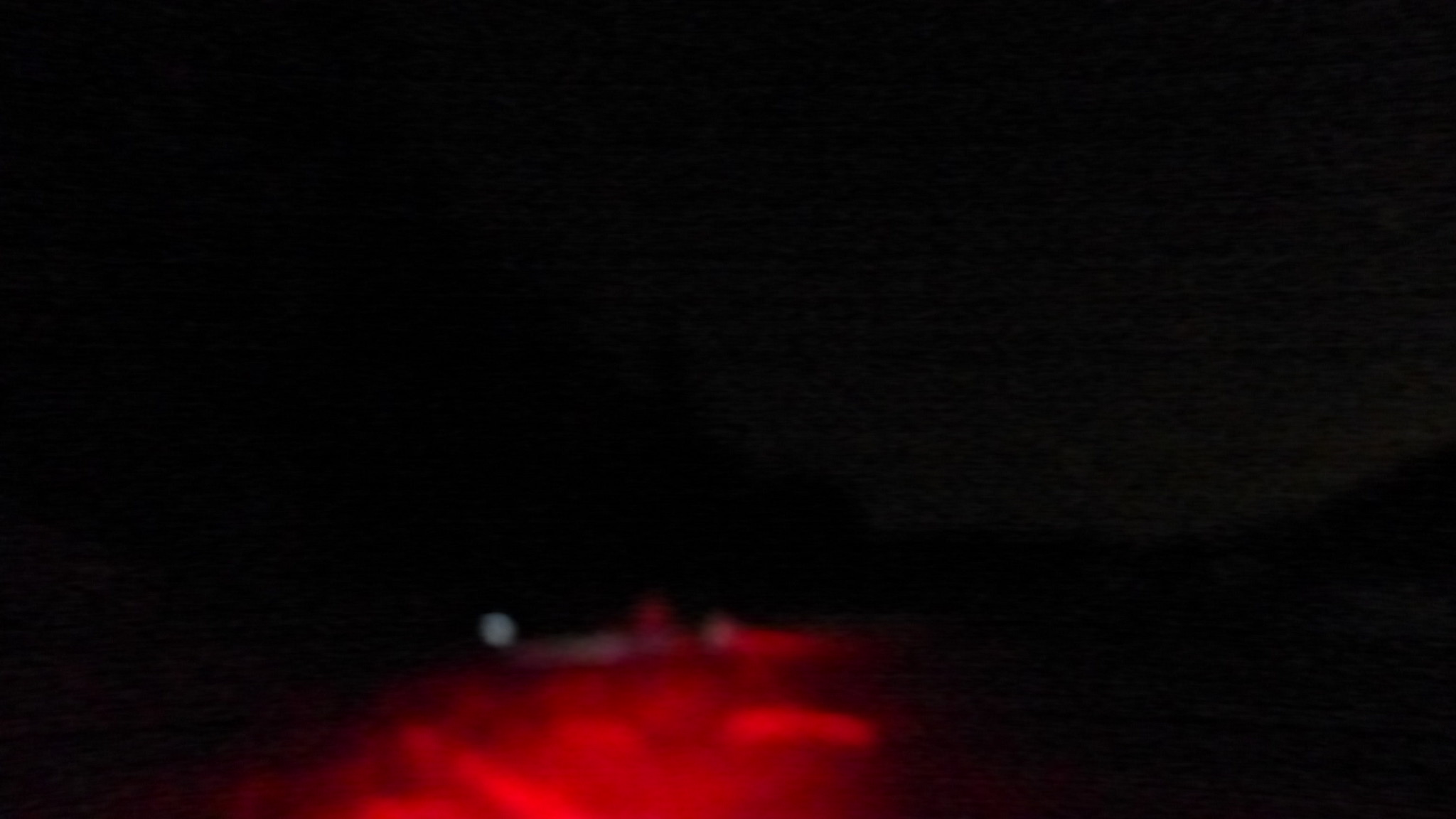The image predominantly consists of a black background, creating a stark contrast that highlights a red object positioned centrally at the bottom of the frame. This red object features a series of darker red lines emanating from it, with two distinct lines branching out to the right side and a couple more extending to the left. Above this central red object, a small, singular white dot is visible. The rest of the image remains devoid of any other distinguishable elements or text, emphasizing the focus on the red object and its surrounding lines.